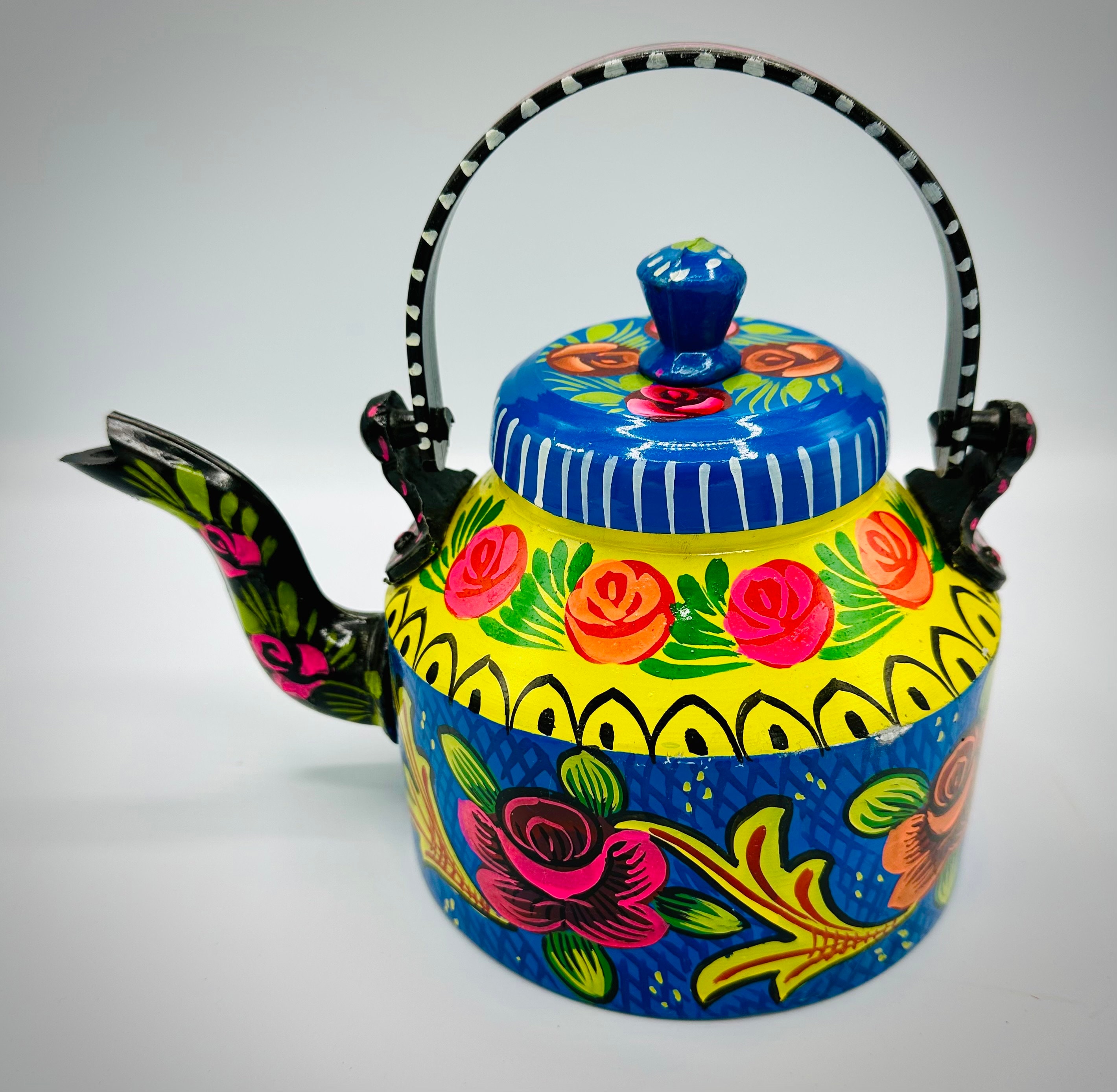A vibrant tea candle sits joyfully in a kitchen setting, instantly captivating with its burst of colors. The handle, designed for easy carrying, is adorned in a striking black and white pattern. The candle itself is a vivid display of blue, white, red, orange, green, lime green, and pink hues. The spout, detailed with green leaves and pink flowers, contrasts beautifully against a black background. The tea candle features intricate designs with pink and orange flowers interwoven with lush green leaves, creating a visually stunning and cheerful atmosphere.